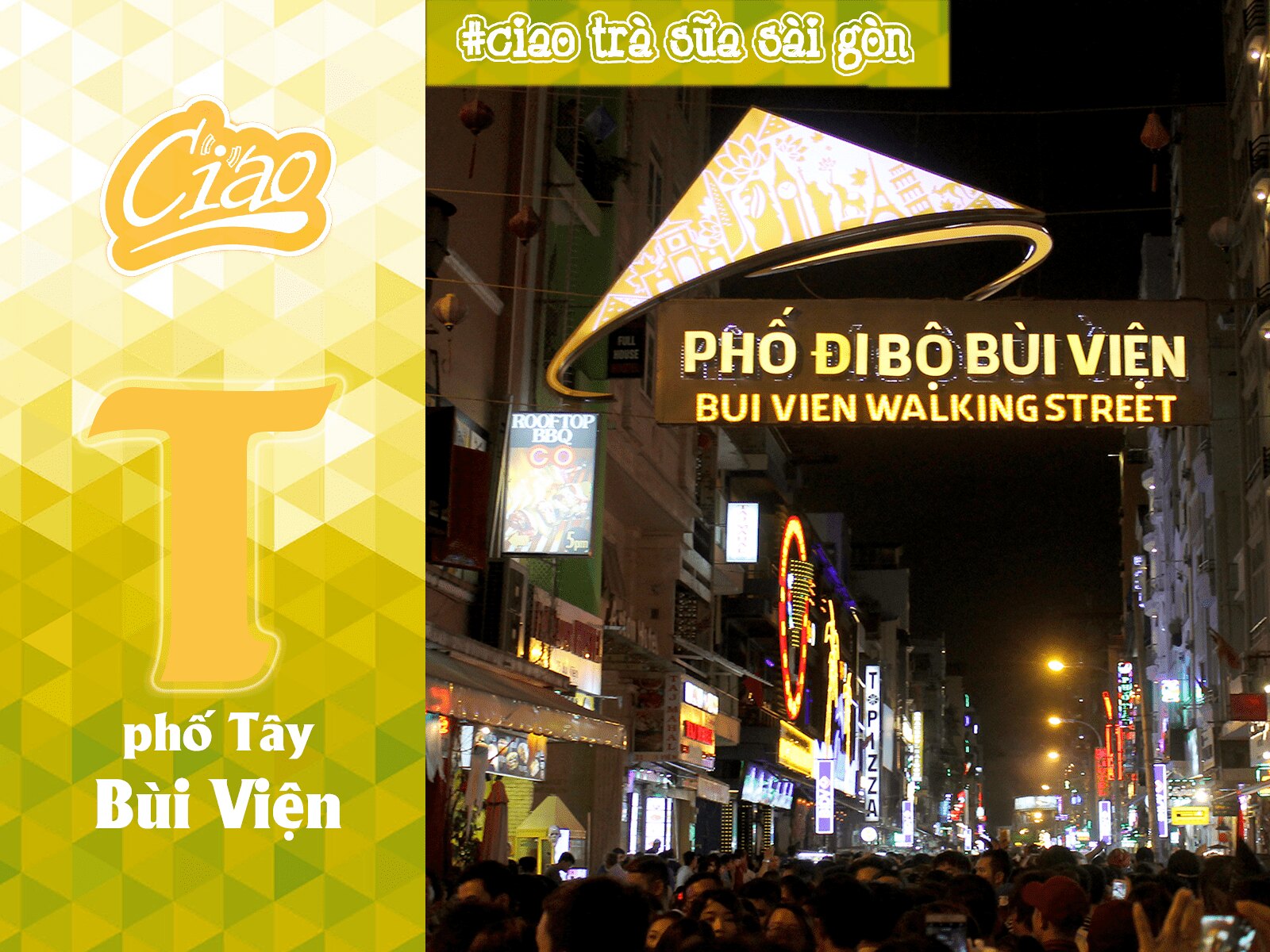The image is a vibrant and bustling city scene, showcasing Bui Vien Walking Street at night. The background is a mix of tall buildings adorned with colorful, illuminated signs that light up the dark sky. The street is packed with a diverse crowd of people, emphasizing the lively atmosphere. Notably, the people appear to be of Asian descent. On the left side of the image, there’s a yellow and green background with the words "Ciao, ti, fo, kei, bui, vien," adding an element of foreign intrigue. The middle right-hand side of the image prominently features the text "Fo Debo Bui Vien Walking Street." At the top, there appears to be additional text in a foreign language on a green rectangle with white letters, along with what looks like a yellow and white cone. Overall, the scene is a vivid portrayal of urban nightlife in an Asian city, full of energy and colorful lights.